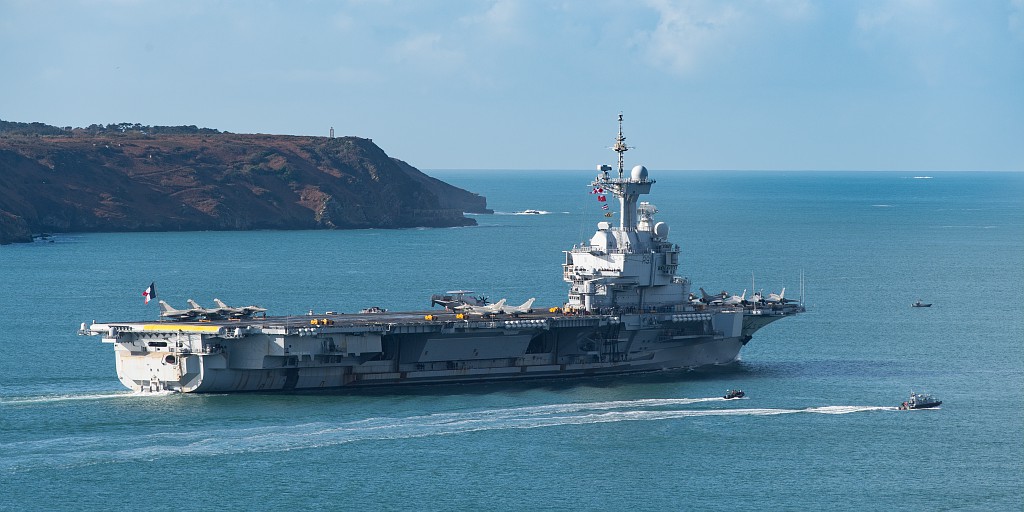The image captures a serene ocean scene under a light blue sky, dotted with wispy white clouds. On the left side of the photo, jagged, rocky cliffs stand out against the horizon. Dominating the center of the image is a large, white military ship, equipped with various military hangars and a satellite. Visible on the deck are approximately ten planes, indicating its role as a transport or landing ship. The ship displays a flag with vertical blue, white, and red stripes, signifying French affiliation. Surrounding the giant vessel are several smaller boats, leaving visible white trails in the calm, blue waters as they speed by. The overall ambiance is of a tranquil yet active maritime scene.